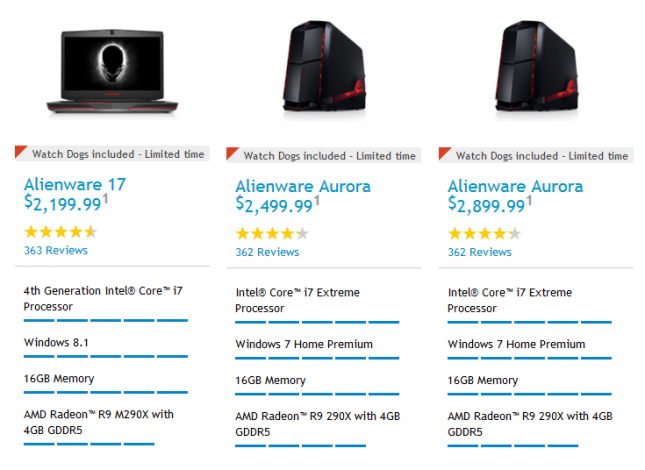The image showcases three items presented in three columns, each enumerating the details and pricing of the respective product, complemented by a picture at the top.

**Column 1:** 
- **Product:** Laptop 
- **Image Description:** An Alienware 17 laptop, opened up and facing the camera, displaying its screen and front part of the keyboard.
- **Details:** 
  - *Special Offer:* Watchdogs included, limited time
  - *Price:* $2,199.99
  - *Rating:* 5 stars from 363 reviews

**Column 2:** 
- **Product:** Desktop
- **Description:** Alienware Aurora
- **Price:** $2,499.99

**Column 3:** 
- **Product:** Desktop
- **Description:** Alienware Aurora
- **Price:** $2,899.99

The columns are designed to give a clear comparison of specific Alienware products, highlighting their prices and key features to assist in an informed purchasing decision.